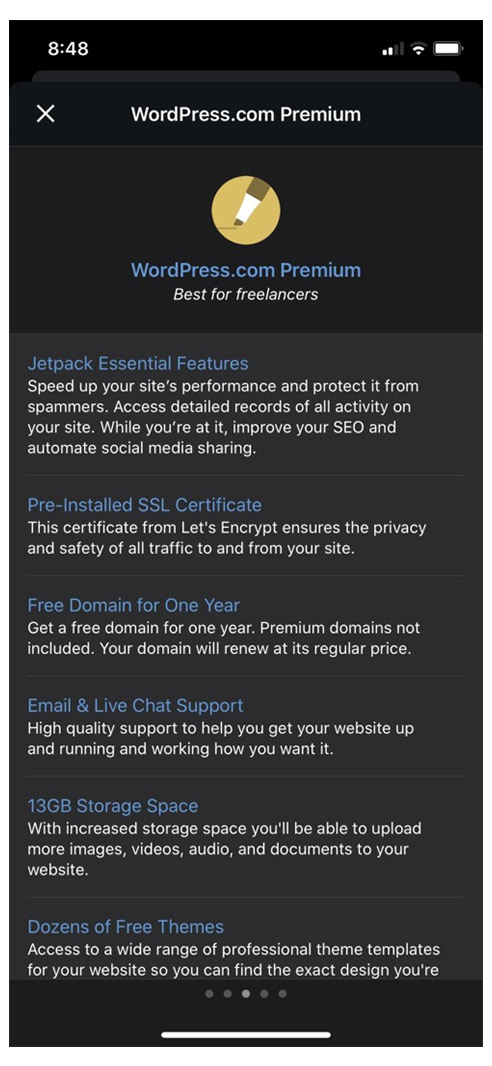The image depicts a smartphone screen in dark mode. At the very top, the current time is displayed as "8:48" in white text. To the right, there are two signal bars, a Wi-Fi icon, and a battery icon. The next line features a white "X" on the left, followed by the text "wordpress.com Premium."

Below this, an icon of a pen writing on a piece of paper is enclosed in a yellow circle. Directly beneath the icon, "Wordpress.com Premium" is written in blue text against the black background. The subtitle "Best for freelancers" appears below this.

The screen contains six paragraphs of information detailing the features of the premium service. The first feature highlighted in blue text is "Jetpack essential features," followed by white explanatory text. Next, "Pre-installed SSL certificate" is in blue, succeeded by additional information. The subsequent entries are "Free domain for one year," "Email and live chat support," "13 GB storage space," and "Dozens of free themes," all presented in blue text and accompanied by descriptive white text.

At the bottom of the screen, there are five horizontally aligned dot indicators and a white bar.